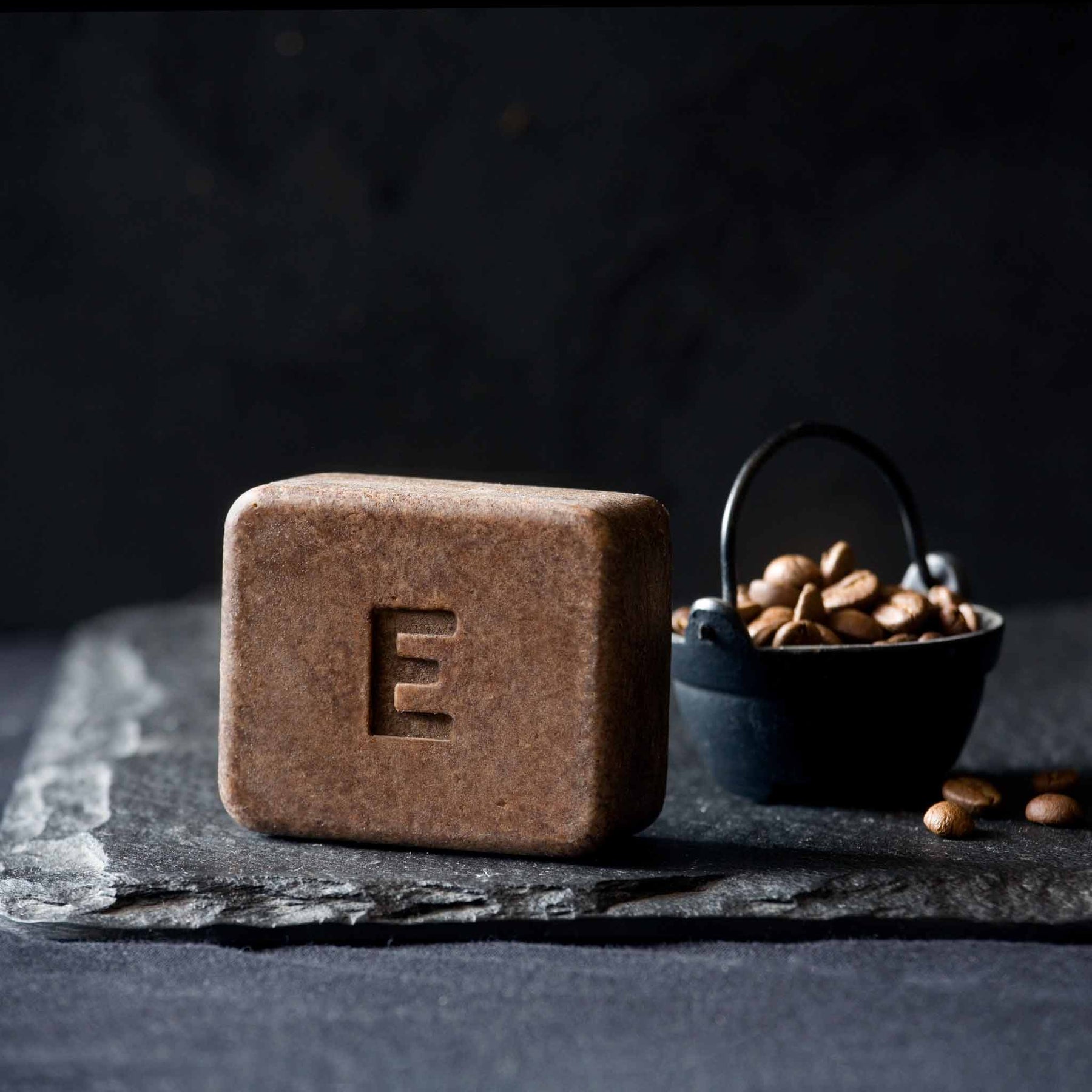This is a professionally taken photograph, likely intended for advertisement, featuring a carefully arranged scene with dark tones. In the foreground, there is a large brown block with chamfered edges and a single capital letter "E" imprinted on its surface. The material of the block is unclear but it resembles a bar of soap. The block rests on a thin, charcoal-colored stone slab, possibly granite or slate, set against a completely black background. Behind the block, slightly to the right, is a small black metal miniature pail, akin to a cast-iron cauldron, filled with lightly roasted coffee beans. A few coffee beans are scattered on the stone slab, enhancing the visual connection between the block and the beans, suggesting that the soap might be coffee-scented or contain coffee grounds. The lighting is directed from the left, casting shadows to the right, which adds depth and highlights the texture of both the soap and the coffee beans.